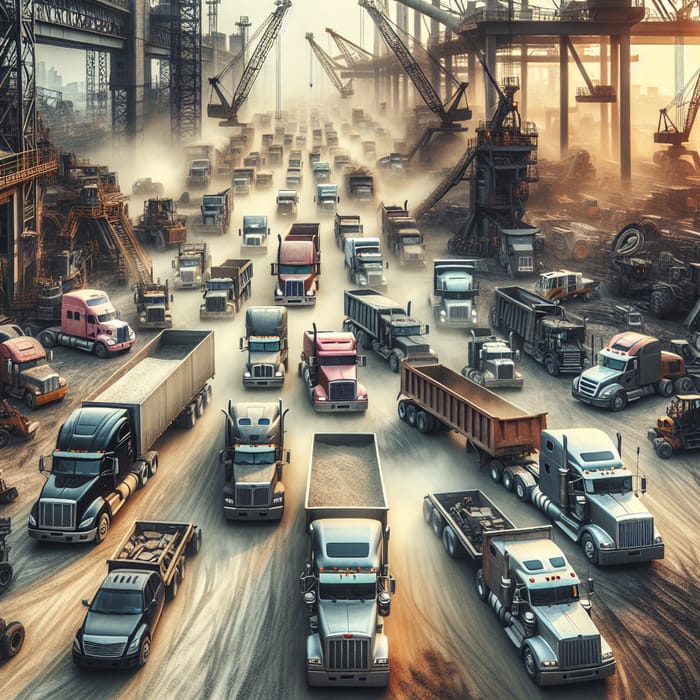The image is an intricate, AI-generated painting of a bustling, imagined industrial city. The scene captures a dynamic fleet of trucks navigating a makeshift dirt road flanked by heavy construction sites. The road, lined with row upon row of trucks, appears to have organically developed lanes formed by the movement of these vehicles. On either side, cranes loom large, busy at work loading and unloading varying cargos into the trucks. Some cranes focus on the lower part and right side of the image, where trucks are backed up into loading docks and rows of parked trucks await their turn. The cargo ranges from sand and dirt to wood, with the focal point being a prominent truck in the center bearing a large, sand-filled trailer. On the right, amid more cranes and structures under construction, there are piles of tires and an array of different truck types, including one peculiar, golf cart-like vehicle. Smoke and debris fill the air, adding to the frenetic energy of this industrial landscape.